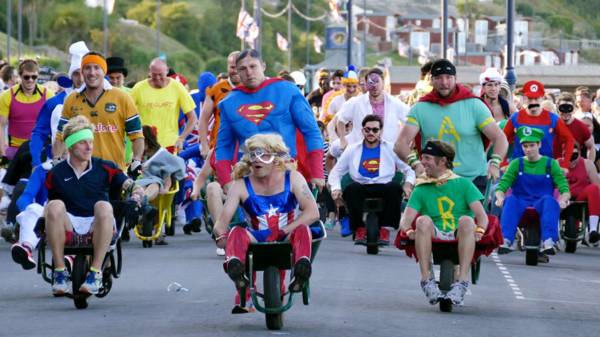The photograph captures an outdoor event, held during the day, where numerous adults dressed as characters from comic books and video games are participating in a playful race. The scene is lively and colorful, set on a paved gray road bordered by greenery on the left and buildings on the right. In the foreground, several pairs of people are racing with one person pushing another in a wheelbarrow.

On the left, a person in a sports uniform, featuring an orange headband and a yellow and green jersey, is pushing someone dressed in a blue and red jersey with a green headband. Next to them, a man in a Superman costume is pushing another man who wears a blonde wig, a light eye mask, and a red, white, and blue dress. 

To the right, another participant, donning a red cape and a green shirt with a yellow emblem, is pushing a person dressed in a yellow cape with a green shirt emblazoned with the letters "DN". Further back, iconic characters like Mario pushing Luigi and a doctor with a "super masher" emblem are also visible. The overall atmosphere is festive, with a diverse group of adults enthusiastically engaging in the fun activity against a backdrop of trees and distant buildings.